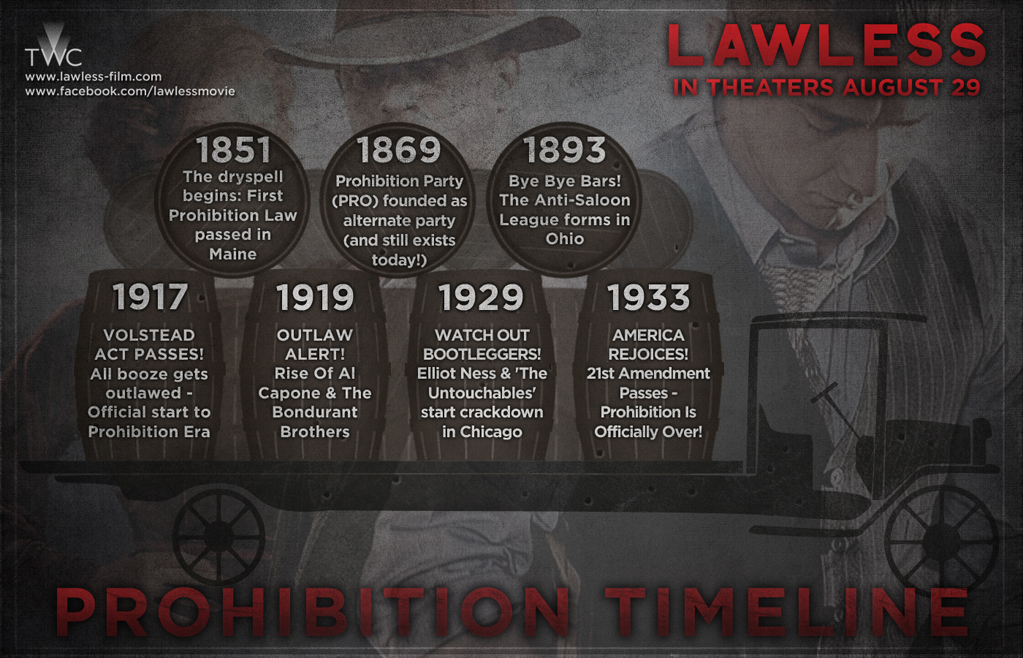The image is a detailed promotional infographic for the film "Lawless," set to be released in theaters on August 29th. The background features a gray Prohibition-era styled photo depicting men in uniforms and ties. In the top left corner, the production company TWC is mentioned along with two websites: www.lawless-film.com and www.facebook.com/lawlessmovie. The top right corner prominently displays "Lawless in theaters August 29th" in red text.

Central to the infographic is a visual representation of a timeline mounted atop an old-timey car, using barrels to illustrate key events in the Prohibition era. The timeline starts with "1851: The dry spell begins, first Prohibition law passed in Maine," followed by "1869: Prohibition Party (PRO) founded as an alternate party, still exists today," "1893: Bye bye bars, the Anti-Saloon League formed in Ohio," "1917: Volstead Act passes, all booze gets outlawed, official start of the Prohibition era," and "1919: Outlaw alert, rise of Al Capone and the Bondurant Brothers." The timeline continues with "1929: Watch out bootleggers, Elliot Ness and the Untouchables start crackdown in Chicago," and concludes with "1933: America rejoices, 21st Amendment passes, Prohibition is officially over." At the bottom, the text "Prohibition Timeline" is highlighted in red.